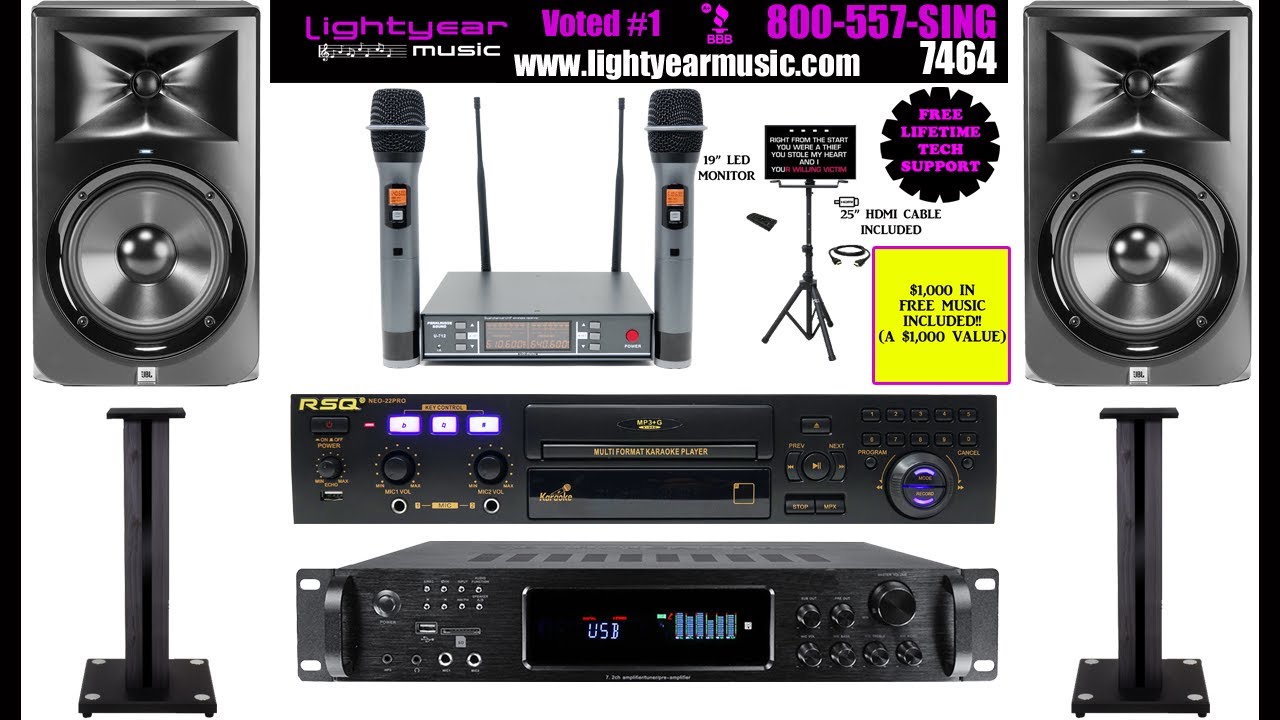This is a detailed advertisement poster set against a solid white background, prominently featuring audio equipment. Along the top runs a black banner with bold purple and white text that reads “Lightyear Music Voted Number 1” followed by “800-557-SING (7464)” and the website “www.lightyearmusic.com.”

The poster showcases a range of audio components and equipment, with two large black speakers positioned on stands on the left and right sides. Each speaker highlights a big woofer and a tweeter mounted vertically, reminiscent of the mid-century design with intricate details that give them almost an X-shape appearance.

Centrally positioned is an elaborate stereo system composed of various black components. At the top is a CD player that may also function as a radio, laden with numerous knobs and buttons. Directly below it, there's a rack-mounted amplifier featuring holes for mounting, multiple control knobs for adjusting volume and tone, and digital screens indicating sound levels. Highlighted text “RSQ” suggests a potential brand name for the stereo components.

Underneath that are two microphones with yellow on-off switches and a compact receiver nestled between them featuring dual black antennas. Adjacent to these microphones is a horizontally-aligned LCD monitor mounted on a tripod, described as a 19-inch LED monitor.

Further adding value to the advertisement, a bright yellow box announces "FREE LIFETIME TECH SUPPORT" and "$1,000 in FREE MUSIC INCLUDED," emphasizing the promotional offer with red and blue linings around the text.

Lastly, small symbols and detailed descriptions scatter across the various audio equipment images, including remote controls and cables, all meticulously designed to advertise Lightyear Music’s electronics store and its products comprehensively.